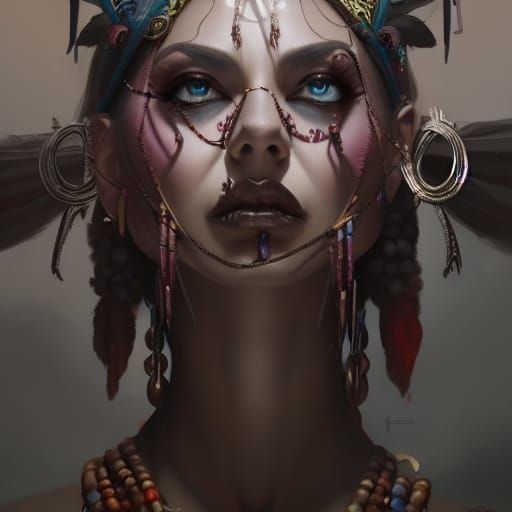In this vertical rectangular image, which appears to be a dark 3D illustration, a woman, possibly stylized in an Eastern Indian or Native American fashion, is depicted from the top of her forehead to just below her neck. She faces the viewer, her light blue eyes gazing upwards. Her pulled-back hair features a headpiece with partially visible black satin bows and various items hanging. Silver, hollow disc-shaped ornaments with hanging elements dangle from each side of her head, and long feathers protrude from just behind her ears. Her face is adorned with intricate jewelry, including facial chains looping over her nose and under her bottom lip, decorated with additional beaded chains and ornaments. She wears multiple strands of necklaces in cream, orange, and blue colors, which end just as the frame cuts off. The background transitions through a gray-beige gradient, enhancing the fantasy style of this computer-generated art. Despite the form taking cues from traditional cultural outfits, the overall scene is fantastical and richly detailed with a combination of make-up, facial jewelry, and elaborate accessories.